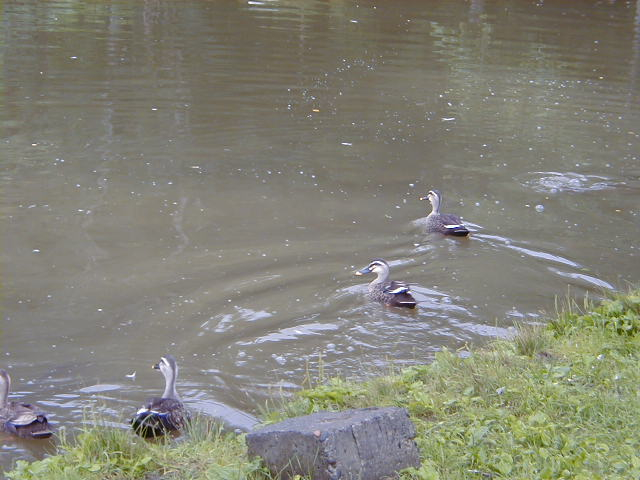This realistic photograph, taken outdoors during the day, features a large body of murky, light brown water, resembling a pond or lake, that occupies the majority of the top left area of the horizontal frame. The water surface is dotted with ripples and small white debris. In the bottom right corner, there is a patch of short green grass interspersed with other green plants. Centrally positioned at the bottom is a rectangular gray stone or cement block, roughly 10 to 12 inches long and about 6 inches high. In the water, starting from the bottom left and swimming towards the top right, are four ducks. These ducks have light brown to gray backs, dark brown and white feathers, and light gray heads with a touch of white around their eyes. They sport dark beaks with slight orange tips and are all facing away from the viewer, creating gentle movements in the water as they sail away from the grassy bank.